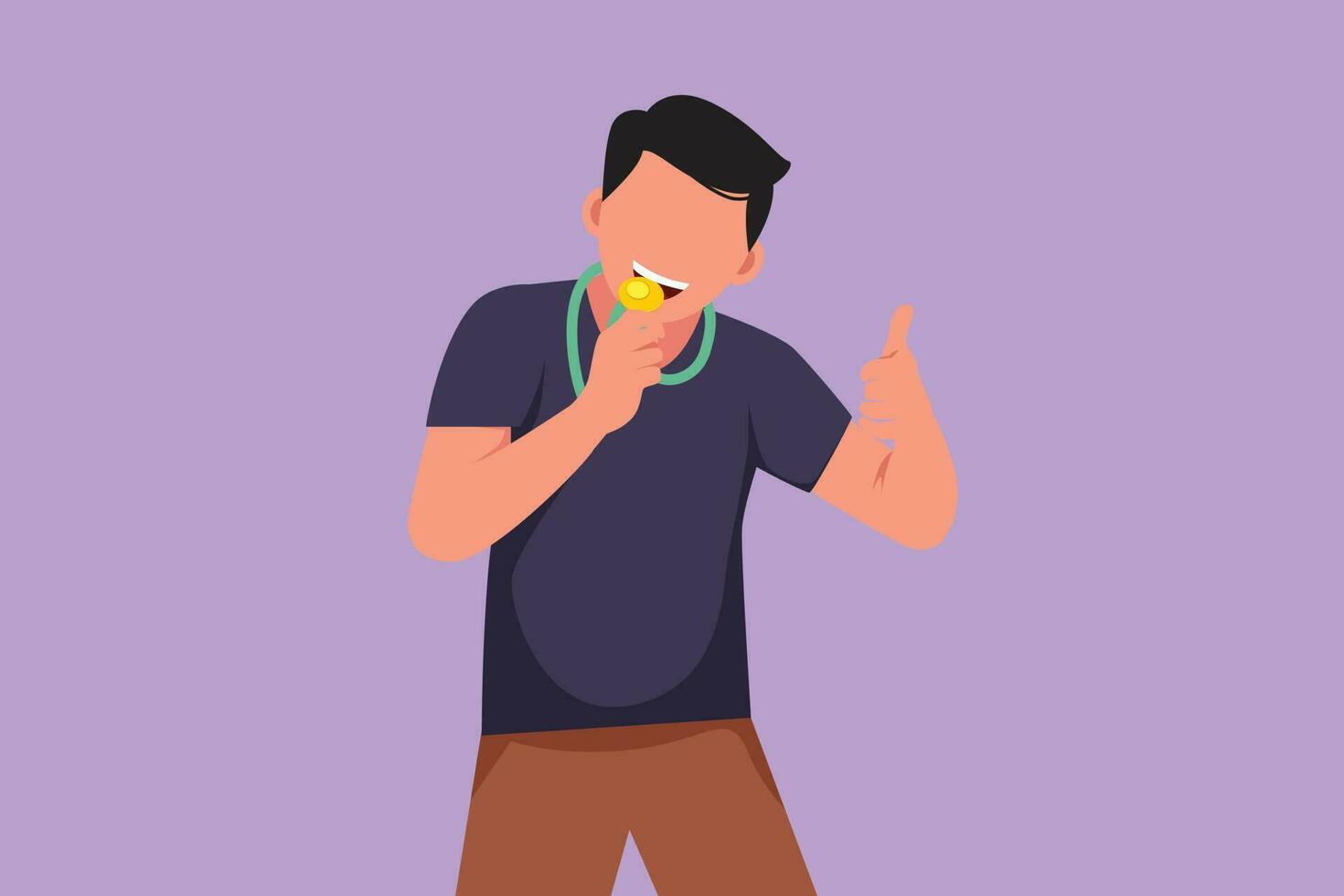This vibrant clipart image features a cartoon doctor set against a lilac purple backdrop. The doctor, who has light skin and short black hair parted to the right, is depicted with a simplified facial design, showing only a mouth with white teeth and two ears, without any nose or eyes. He is dressed in a navy blue short-sleeved t-shirt and brown pants. The doctor holds a gold medal with a light green band in his right hand, which he is biting between his teeth while giving a thumbs up with his left hand. Shadows are cast on his shirt and pants, adding depth to his figure. The scene is lively and colorful, with attention to detail in the doctor's posture and expression.